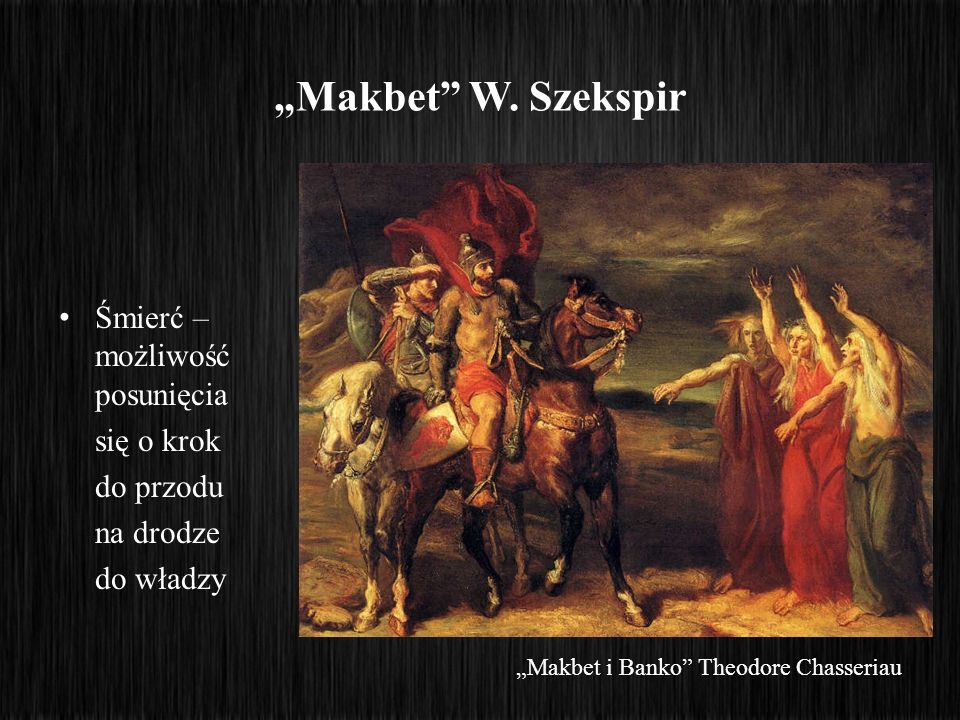The image is a detailed painting predominantly in golds, earth tones, and deep reds, set against a grainy black background. At the top, it features the word "Macbeth" in quotation marks, followed by what appears to be a stylized version of "W. Shakespeare" written as "W.S.C.E.K.S.P.I.R." or "W. Spexper." The painting itself depicts an outdoor scene, possibly from the 16th to 18th century. In the top section, three soldiers dressed in Roman or Greek-inspired armor ride horses—one bronze, one white—one of the riders has a flowing red cape. To their right are three women who resemble witches: one woman has her hair covering her bare chest and a skirt pulled down, another has her hands raised wearing red, and the third, dressed in brown, has her arm extended to the right. The sky behind them is dark and ominous. Adjacent to the painting on the left side is a list of names in white text, likely written in Polish, including Smirik, Mosolowicz, Posniecka, C. O'Croke, D. Przodko, N. Drodza, and D. Wladlejczyk. Below this list, it reads "Macbeth Ebenko by Theodore Chassereau" in white letters.